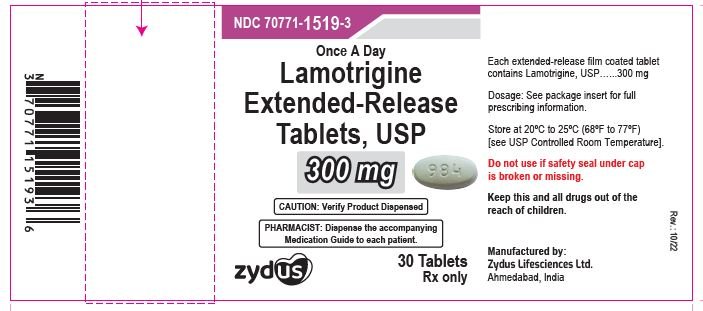This image illustrates a flat, detailed diagram of a prescription medication box, resembling the printed design one would see before it is folded into the shape of a box. The layout is presented as a horizontal rectangle with a purple outline. Dotted purple lines and an arrow indicate where the box should be folded and how the interior flap should be positioned.

On the left-hand side of the diagram, there is a vertically-oriented barcode with the number "7077115193". On the right-hand side, the following text is prominently displayed: "Once a day Lamotrigine Extended-Release Tablets USP 300 mg". Below this, there is an illustration of an oval-shaped pill with the number "984" imprinted on it.

Further text advises: "Caution: Verified product. Dispense accompanying medication guide to each patient." It also includes several pharmacy logos, specifically "Zydus". The notation "30 Tablets Rx Only" is also present, signifying the prescription-only status and quantity of the medication. In the upper left-hand corner, the National Drug Code (NDC) is displayed in purple with white text: "NDC 70771-1519-3".